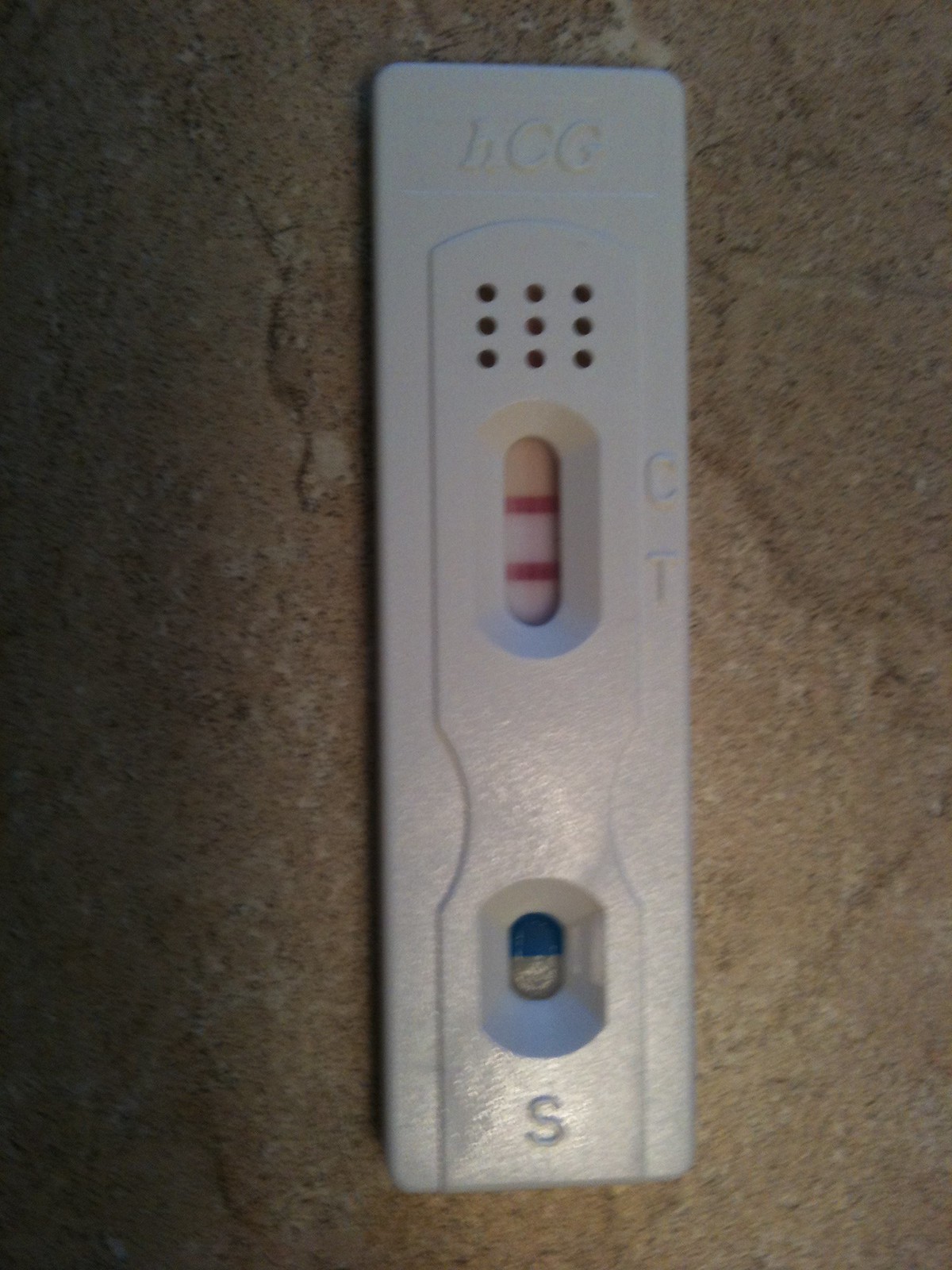The image depicts a white pregnancy test resting on what appears to be a faded brown surface, possibly concrete or rock, though it could be a countertop. The test is labeled with "HCG" at the top in cursive letters. Below this, there are nine small circles. Further down, the test has labeled sections with "F" at the bottom and "C" and "T" in the middle, presumably standing for Control and Test. The central white display area shows two red lines, indicating the results. The bottom section of the test has a divided area, half clear and half blue. This detailed description emphasizes the test's purpose and elements to determine a positive or negative pregnancy result.